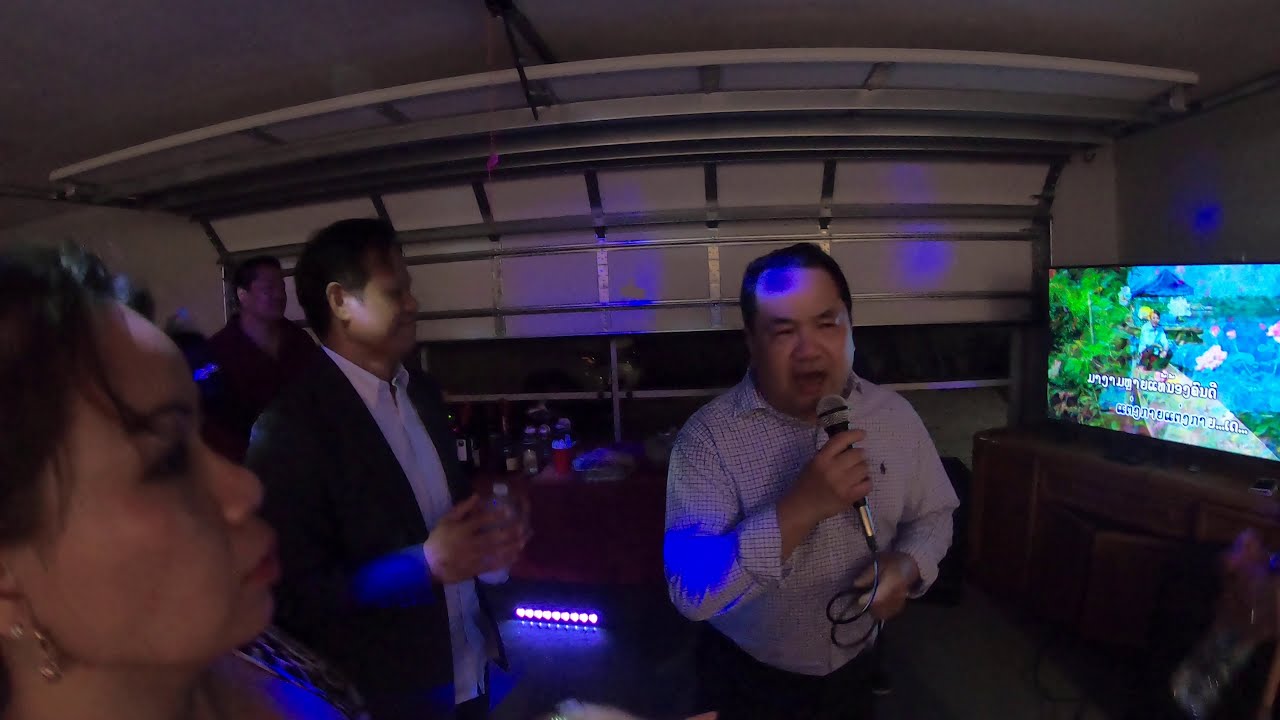A group of four individuals, likely of Asian or Indian descent, are gathered in what looks like a home garage or a private karaoke bar, complete with an indoor bar setup. Despite the dim lighting suggesting it's nighttime, the setting is cozy with white walls and a hint of a sliding garage door in the background. The central figure, a middle-aged man in a patterned checkered collared shirt, passionately sings into a microphone, holding a water bottle in his other hand, and is deeply engaged in the karaoke performance. To his left, a woman with short black hair looks on, while a man in a suit and another in a black collared shirt complete the group of onlookers. A brightly lit TV screen on the right side of the image displays colorful visuals and foreign language lyrics, enhancing the lively atmosphere as everyone enjoys the moment.